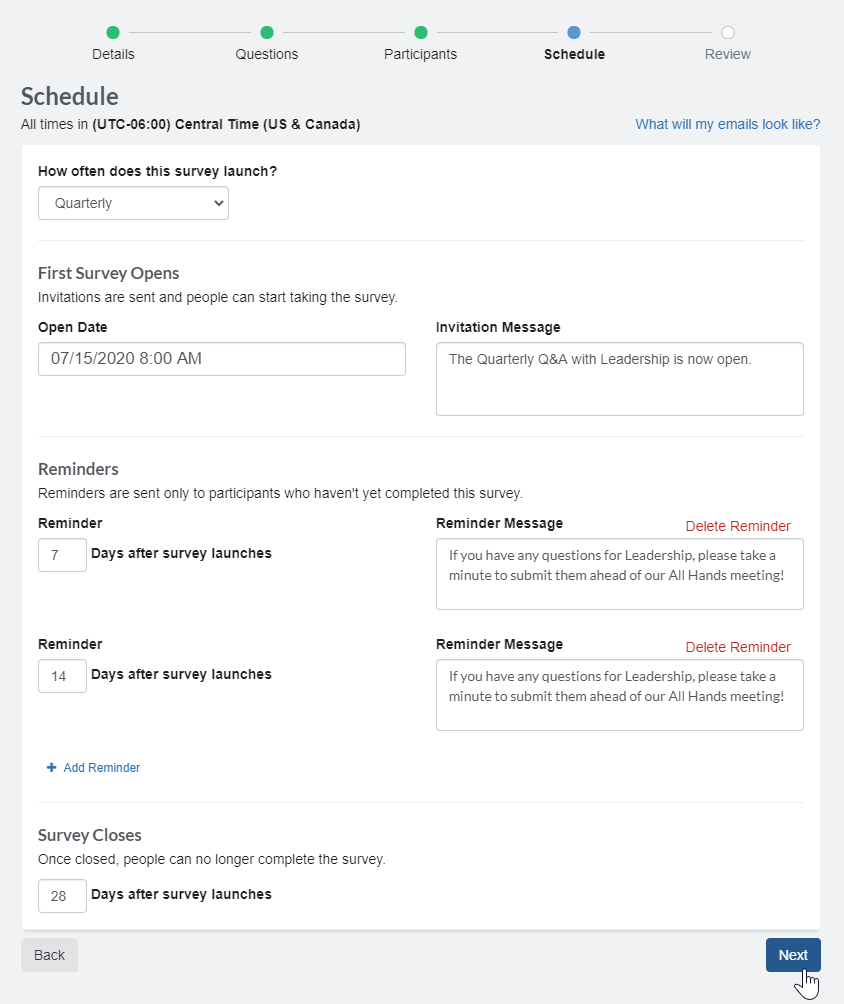This image is a screenshot of a section of a website featuring a light gray background, with a centrally positioned white rectangle inset from the edges. At the top of this white pane, there are five evenly spaced dots stretching across the width of the page. The first three dots are green, the fourth dot is blue, and the fifth dot is white with a thin light gray outline. Thin medium gray lines connect these dots. Below each dot, there is text: black for the first three, bolded black under the blue dot, and light gray under the last dot. The text reads, from left to right, "Details," "Questions," "Participants," "Schedule," and "Review."

Lower down and to the left, the word "Schedule" is displayed in large dark gray text. Beneath this heading, a line of small black text reads, "All times in," followed by bolded text within parentheses, "UTC-0600," and further specifications in bold, "Central Time," and in parentheses, "U.S. and Canada." To the right, there is small blue text asking, "What will my emails look like?"

In the top left of the white pane, bolded black text poses the question, "How often does this survey launch?" Directly below this, a white dropdown menu with a thin medium gray outline has "Quarterly" written in black text on the left and a dark gray downward caret on the right. Beneath this dropdown, a thin light gray line spans almost the entire width of the pane, separating it from the lower section.